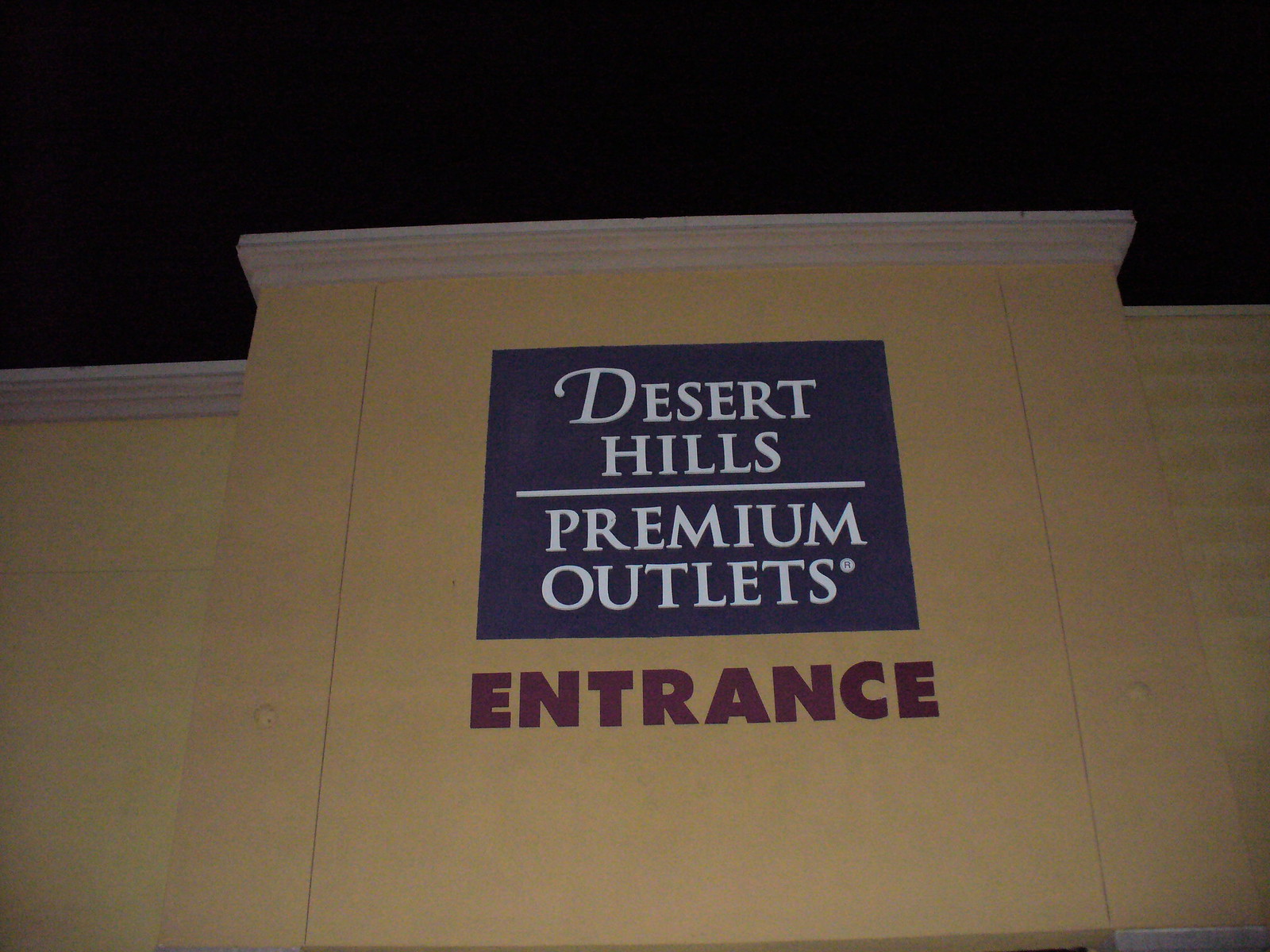The image captures the top portion of a sand-colored (or custard yellow) stucco building, part of an outlet mall, taken at nighttime against a black sky. The structure features a white decorative trim along the top, just below the rooftop. The focal point is a prominent sign in the center with a navy blue background and white uppercase letters reading "DESERT HILLS PREMIUM OUTLETS." Below this, in bold red capital letters, is the word "ENTRANCE." The section with the sign protrudes slightly from the main building. On the very bottom right of the image, a small part of the doorway to the entrance is visible, suggesting that it continues below the frame. The attention to detail in the sign and trim, along with the nighttime setting, highlights the entrance to this upscale mall.